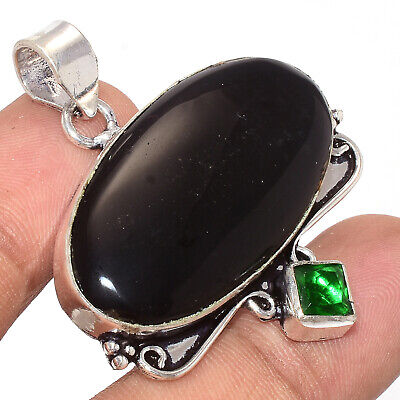This color photograph captures a close-up view of two human fingers holding a piece of jewelry against a neutral backdrop. The jewelry features a prominent, smooth oval cabochon in pitch black, encased in a metal band. Below the main stone sits a smaller, diamond-shaped green gem, possibly an emerald, adorned with three small silver beads and delicate filigree work on either side. The piece includes a silver hook at the top, suggesting it is designed to be a pendant for a necklace or bracelet. The image is detailed enough to show the texture and placement of the fingers, which hold the jewelry delicately, emphasizing its approximate size—the length of two finger joints.